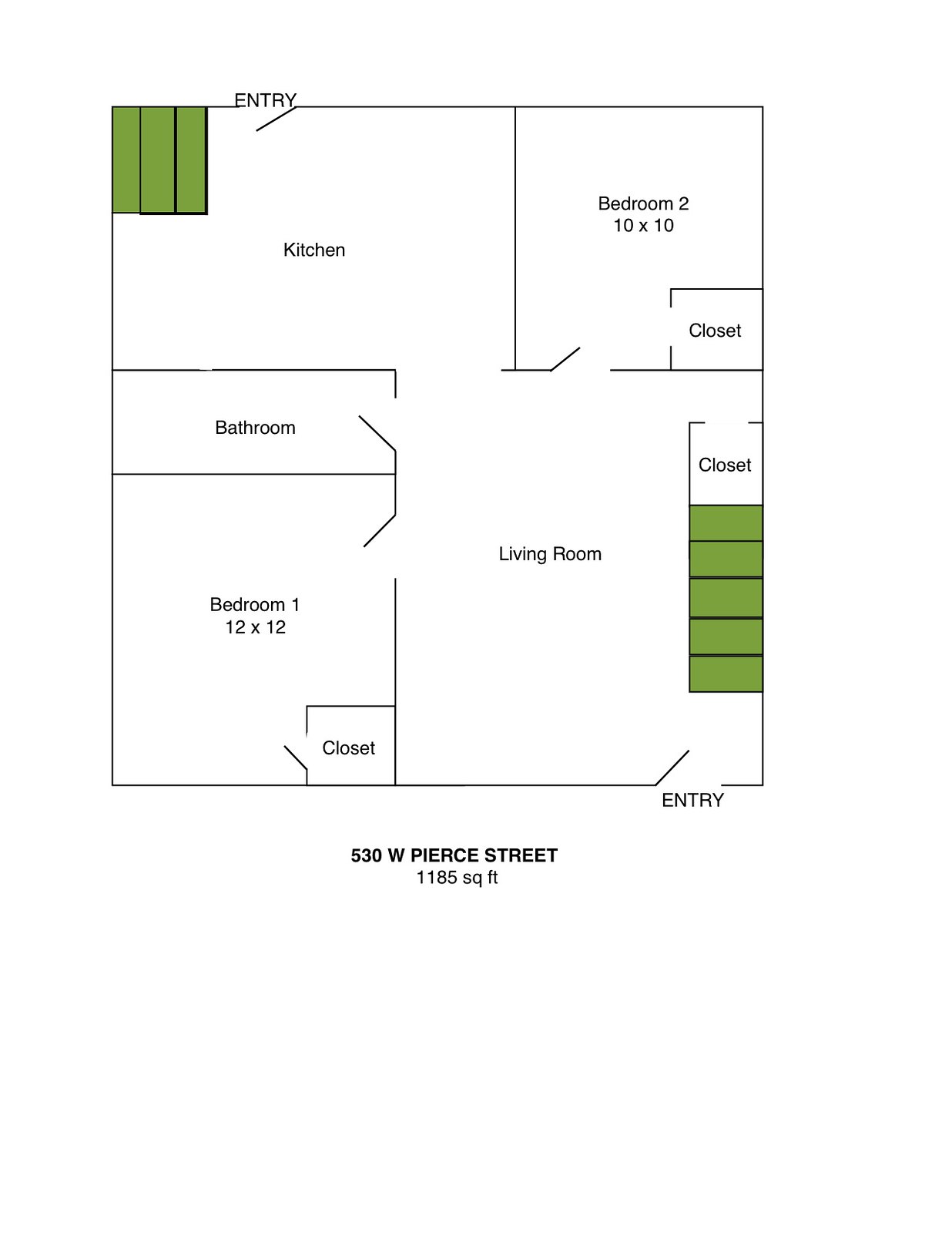The image depicts a meticulously designed floor plan rendered with precision, likely using a 3D modeling software. The floor plan features a white background with clearly defined black lines delineating each section of the space. The layout presents various labeled areas, each meticulously detailed:

- **Top left:** The entry point is indicated, accompanied by a door symbol. Beside the entry, there is a green square with lines inside it.
- **Central area:** Moving downward from the entry, the layout transitions into the kitchen area, followed by the living room. On the right side of the living room, a closet is depicted, adjacent to more green squares.
- **Bottom right:** The word “ENTRY” is also present, suggesting an additional point of entry.
- **Left side:** The top portion features the bathroom. Below the bathroom, Bedroom 1 is marked, measuring 12 by 12 feet, complete with a small box symbolizing a closet and a door.
- **Top right:** Bedroom 2 is indicated, measuring 10 by 10 feet, with a designated closet space illustrated by a small box.

At the very bottom of the image, the address "530 W Pierce Street" is noted, along with the total area of "1185 square feet," giving a clear sense of the overall size and layout of the property.